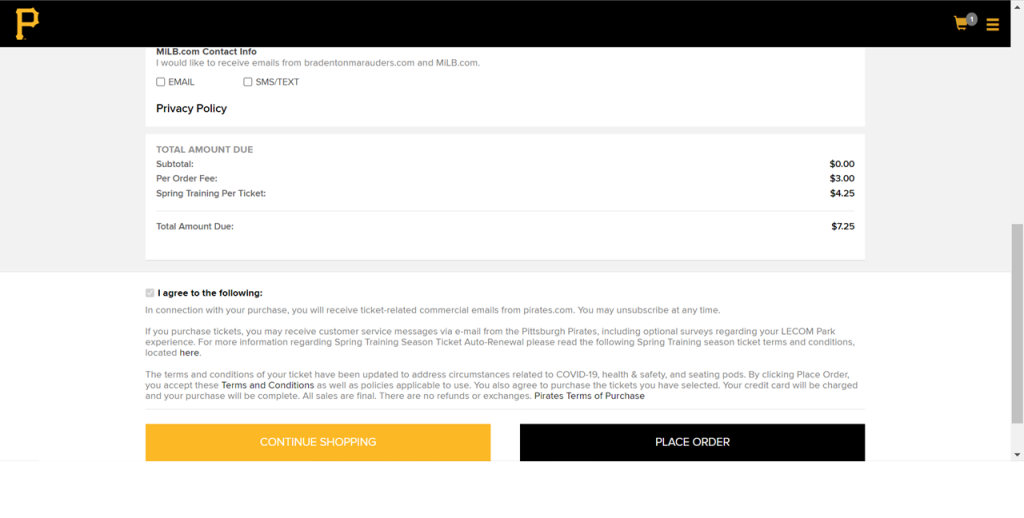The image depicts a website interface dedicated to purchasing tickets for Pittsburgh Pirates games, specifically for spring training. 

In the upper-left corner, there is a prominent yellow letter "P" designed in the signature font style of the Pittsburgh Pirates. The top toolbar, set against a black background, features a small yellow shopping cart icon on the upper right. This cart includes a grey circle with the number "1" inside, indicating there is one item in the shopping cart. Adjacent to the cart icon are three horizontal lines stacked on top of each other, representing a dropdown menu for additional navigation options.

The page's main body is set against a grey background and contains several white informational boxes. The first white box displays "MLB.com contact info" with options to choose either email or SMS text for communications; neither of the corresponding checkboxes are selected. Below this, a link labeled "Privacy Policy" is displayed in black text.

Further down, another white box outlines the financial summary for an order with the following details:
- "Subtotal": $0
- "Per Order Fee": $3
- "Spring Training Per Ticket": $425
- "Total Amount Due": $725

This detailed information confirms that the website is primarily used for purchasing tickets to Pittsburgh Pirates spring training games.